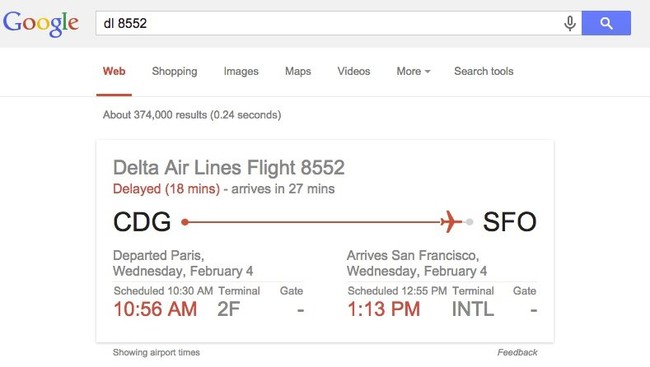The image appears to be an old screenshot of a Google Flights search result page. Along the top, there is a light gray bar featuring the classic Google logo. Below the logo is a search bar with the text "DL8552," accompanied by a microphone icon and a blue button with a white search icon. The search results are displayed beneath this bar, with the "Web" tab selected, highlighted in red with a red underline. To the right, other options such as "Shopping," "Images," "Maps," "Videos," "More" (with a dropdown menu), and "Search tools" are visible in gray.

The search results indicate there are about 374,000 results found in 0.24 seconds. The main displayed detail is for Delta Airlines Flight 8552, listed in gray text. The flight information is highlighted in red, noting a delay of 18 minutes, with an expected arrival in 27 minutes.

The flight originates from Charles de Gaulle Airport (CDG) in Paris and is destined for San Francisco International Airport (SFO). There's a graphical line with a plane icon depicting the flight's path from CDG to SFO. Detailed flight information indicates that the flight departed Paris on Wednesday, February 4th. It was scheduled to leave at 10:30 a.m. but actually departed at 10:56 a.m. from Terminal 2F, with no specified gate (marked with a minus sign).

The arrival information shows that the flight is expected to arrive in San Francisco on the same day, scheduled for 12:55 p.m., but now estimated to arrive at 1:13 p.m. at the International Terminal, with the gate also marked with a minus sign. Below this, there appears to be additional details in gray text that are not readable.